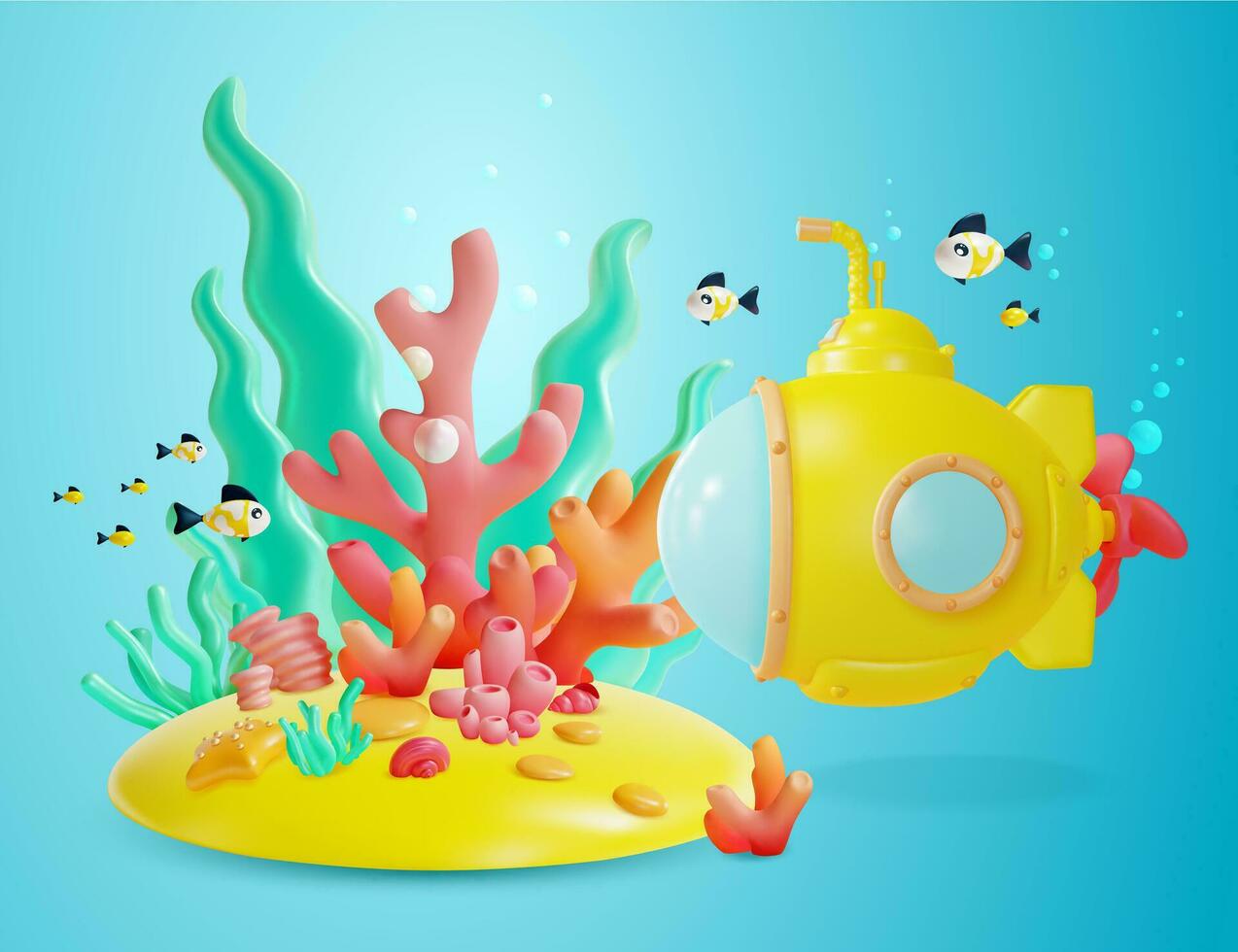This detailed and vibrant image portrays an underwater scene reminiscent of a children's painting or a video game. The backdrop of the illustration is a gradient of dark to light blue, representing the depths and light refractions of underwater. Central to the composition is a yellow submarine, designed with a cartoonish, 3D appearance, featuring round windows at the front and the side, and creating small bubbles as it navigates through the water.

To the right of the submarine, there is a cluster of three fish, predominantly yellow and white, with a tiny all-yellow fish among them. An additional school of fish, composed of similar colors with black fins and tails, swims towards the submarine from the left. The fish are depicted as oval-shaped, adding to the playful aesthetic of the scene.

A coral reef, positioned centrally, boasts a blend of teal and pinkish-red coral formations. The reef is accented with various underwater elements, such as starfish and a snail, nestled in a sandy yellow area likely representing the island’s surface. The overall depiction is set against a bisected foreground of dark blue water transitioning to a white center, emphasizing the scene's depth and whimsical charm.